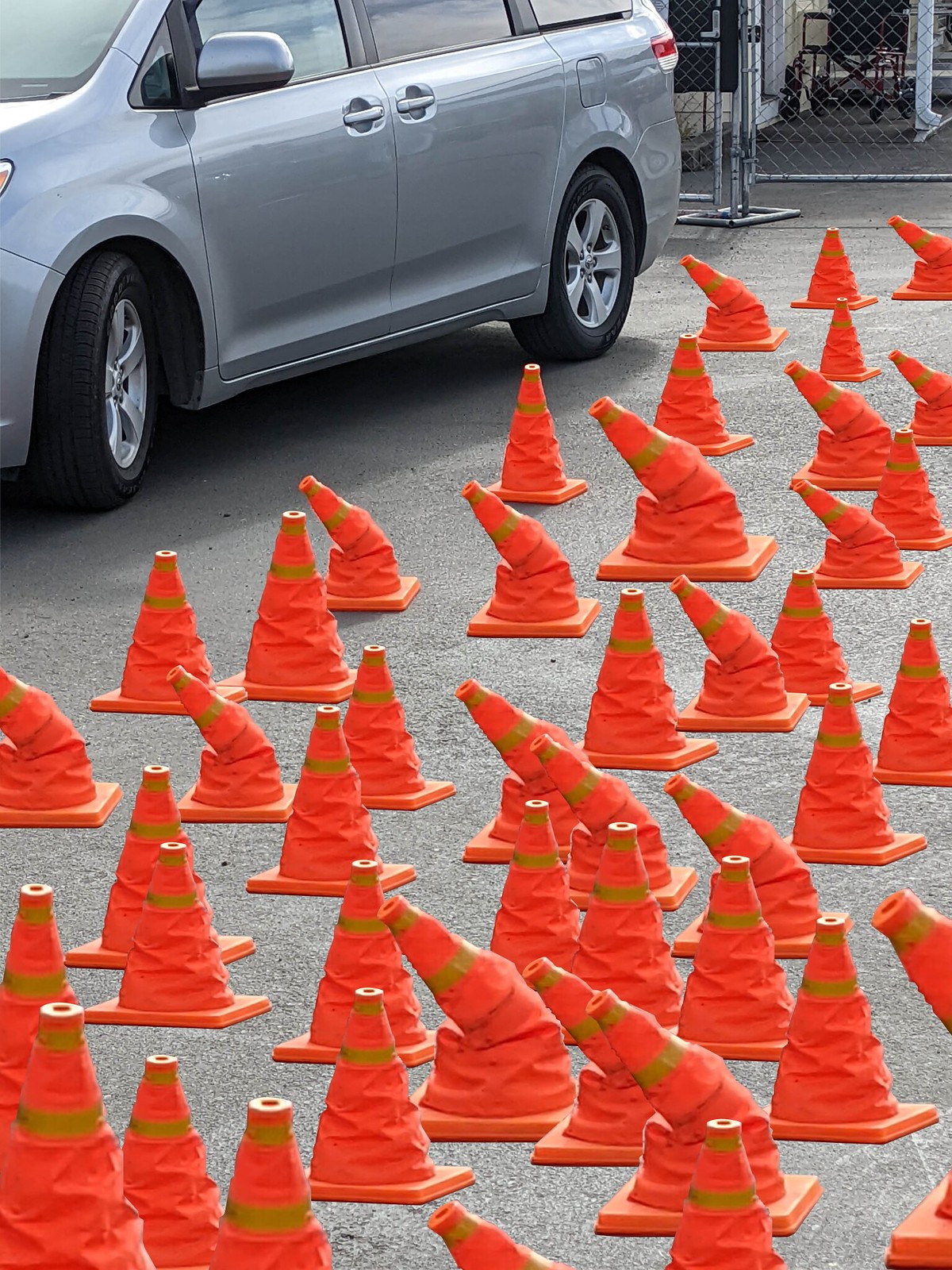This vibrant daytime photograph features an expansive asphalt area dominating the scene. In the upper left quadrant, the right side of a gray minivan is visible, angled downward towards the left. A chain-link fence can be spotted in the back right-hand corner, serving as a backdrop. Scattered throughout the lower half and the entire right-hand side of the image are numerous orange collapsible cones. Some of these cones stand upright while others are bent over towards the left, creating an intriguing texture. The exact nature of the cones is ambiguous, leaving it unclear whether they are genuine physical objects or digitally added elements.